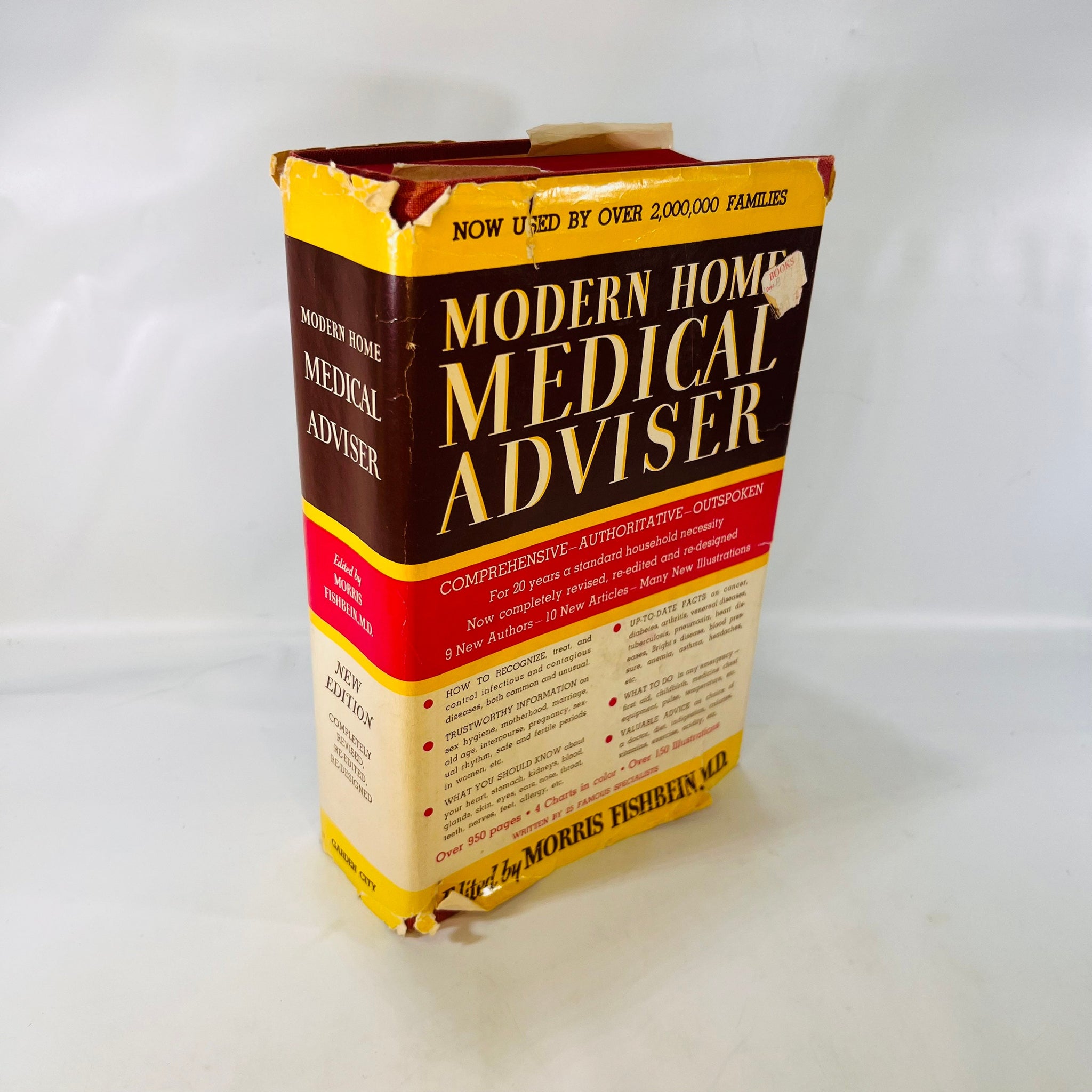A photograph captures an old, worn-out book standing on end against a plain white background, barely casting a shadow. The book's cover and dust jacket are visibly torn and heavily used, suggesting it has been read countless times. The title, "Modern Home Medical Advisor," is prominently displayed in black letters on a yellow banner, which also states "Now used by over two million families." The top of the book cover is slightly ripped. The spine and the front cover reveal more details: a red band running horizontally across the middle that reads "Comprehensive, Authoritative, Outspoken" and additional text, which includes phrases like "for 20 years a standard household necessity, now completely revised, re-edited and redesigned," and mentions of new articles and illustrations. Towards the bottom, a white or off-white section with black text offers further information, including how to recognize trustworthy medical advice. At the very bottom of the book, a yellow banner with black font credits the editor, "Morris Fishbein, MD."